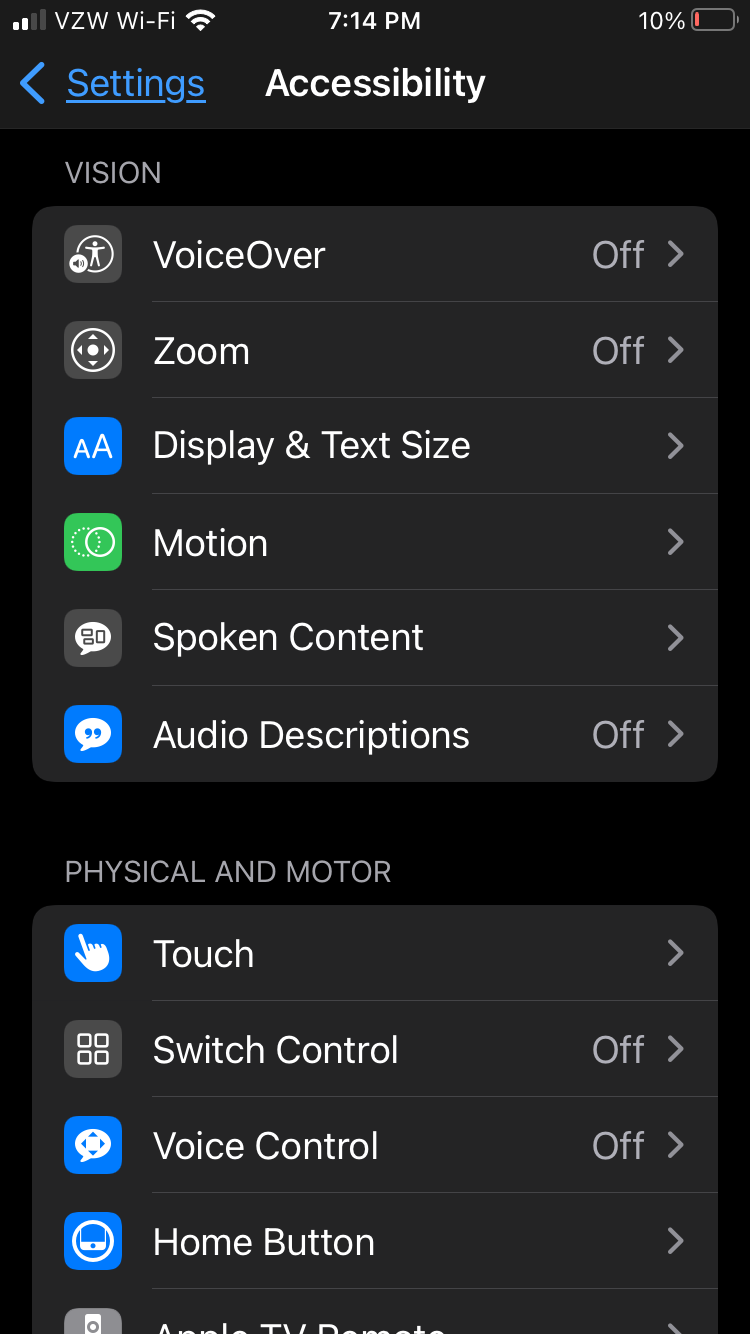The image depicts a vertical cell phone screen with a black background, presenting a detailed view of the settings panel within the accessibility submenu. In the upper left-hand corner, various cell phone icons are displayed, including the Wi-Fi network name "VCW Wi-Fi." The current time, shown centrally at the top, is 7:14 p.m., and the battery indicator in the upper right reveals a low charge at 10%.

The settings panel is specifically focused on accessibility features, highlighting various vision preferences. These include options such as VoiceOver, which is currently off, Zoom, also off, Display & Text Size, Motion, Spoken Content, and Audio Descriptions. Below these options, there are categories for physical and motor accessibility controls, detailing settings related to touch sensitivity, switch control, voice control, and the home button functionality.

The interface does not indicate whether the operating system is iOS or Android, and there is no date visible on the screen. However, it is evident that the device offers a comprehensive suite of accessibility accommodations, providing detailed customization for users with various needs.